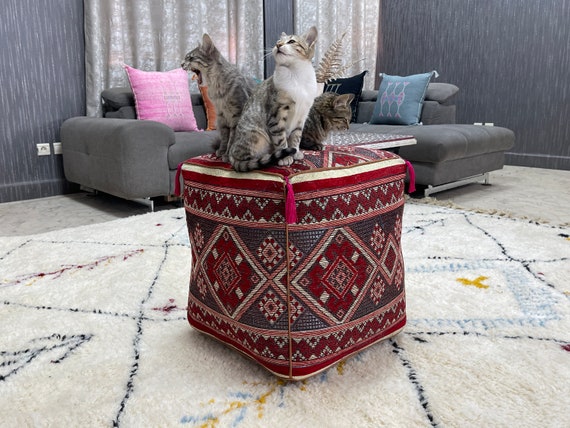In this detailed photograph, we see three cats positioned closely together on an ornate, cube-shaped ottoman. The ottoman, about two cubic feet in size, features a lavish red, white, and maroon diamond pattern and has the appearance of a Persian rug wrapped around a plump, square cushion. It sits prominently in the center of a room on a plush white Moroccan-style rug adorned with black lines and gold and red symbols.

Each cat displays a different behavior: one is yawning, another is lazily lying down as if nearing sleep, and the third is standing up, gazing towards the ceiling. The cats, with coats of light and dark gray accented by patches of white, add to the charming scene.

In the background, the room's dark gray walls with white streaks offer a stylish, contemporary contrast to the colorful ottoman. Above, tan and white curtains frame the upper part of the image. A dark gray couch occupies the center area, decorated with vibrant cushions in shades of pink, red, blue, and light grayish blue, enhancing the overall ambiance of the room.